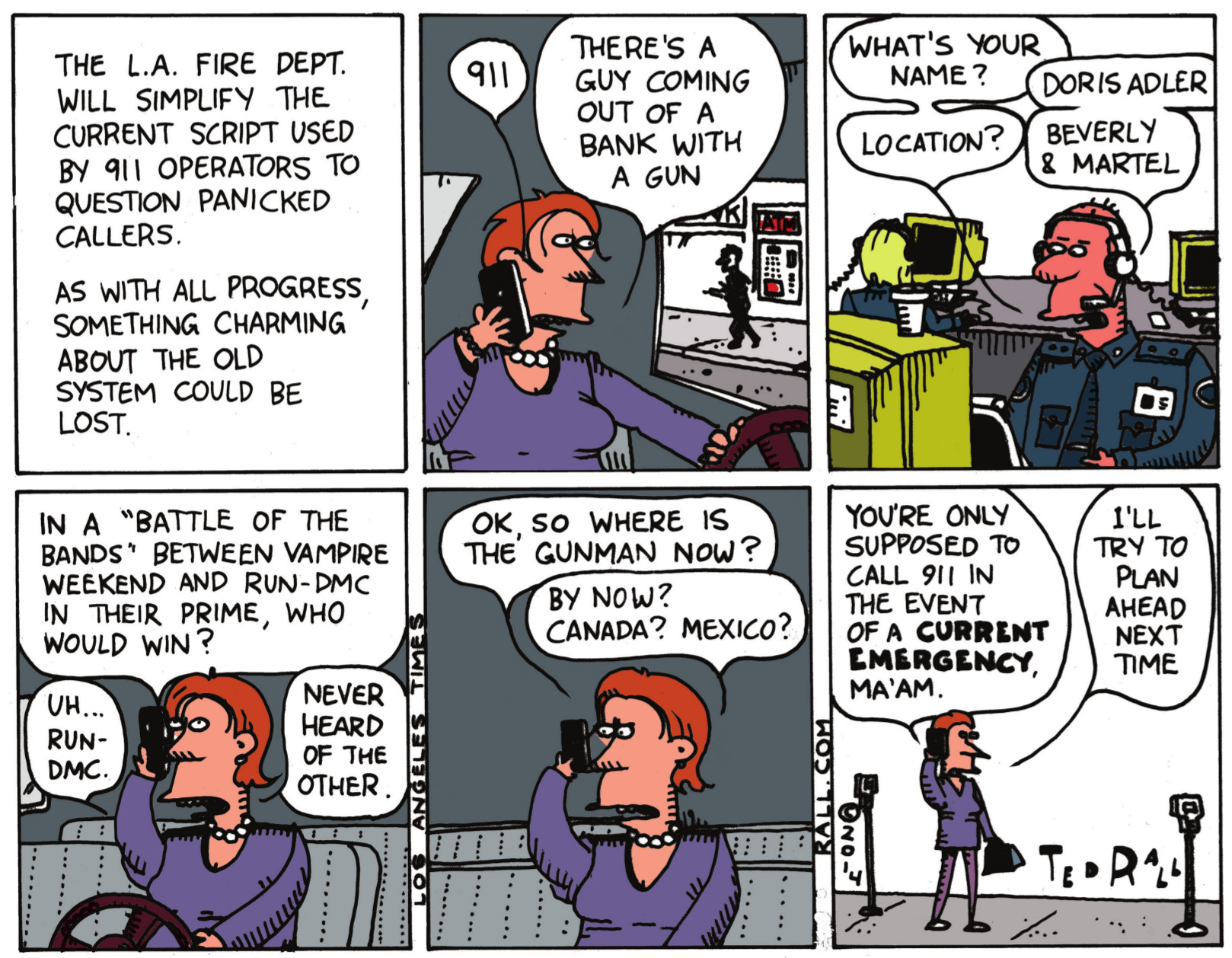This six-panel cartoon, created by Ted Rall and published by the Los Angeles Times and Rall.com in 2014, critiques changes to the 911 call response system. The comic is arranged in two rows of three panels each, with the top left panel containing a text introduction that reads: "The LA Fire Department will simplify the current script used by 911 operators to question panic callers. As with all progress, something charming about the old system could be lost."

The second panel depicts a woman with red hair and a purple shirt, driving her car and dialing 911. The third panel shows a 911 operator answering the call. The bottom row continues the scenario: the woman, now identified as Doris Adler, reports a gunman coming out of a bank. The operator asks a series of increasingly irrelevant questions, including, "In a battle of the bands, between Vampire Weekend and Run DMC in their prime, who would win?" Doris humorously responds that she prefers Run DMC as she hasn't heard of the other band.

By the final panel, Doris is shown having parked her car and standing on the sidewalk between two parking meters, still on the phone with the operator. The interaction concludes with the operator scolding her for not calling with a more immediate emergency, to which Doris wryly responds, "I'll try to plan ahead next time." The strip uses a mix of colors such as white, black, orange, tan, purple, various shades of gray, maroon, and green, underscoring its mock-serious tone while delivering social commentary on bureaucratic inefficiencies.